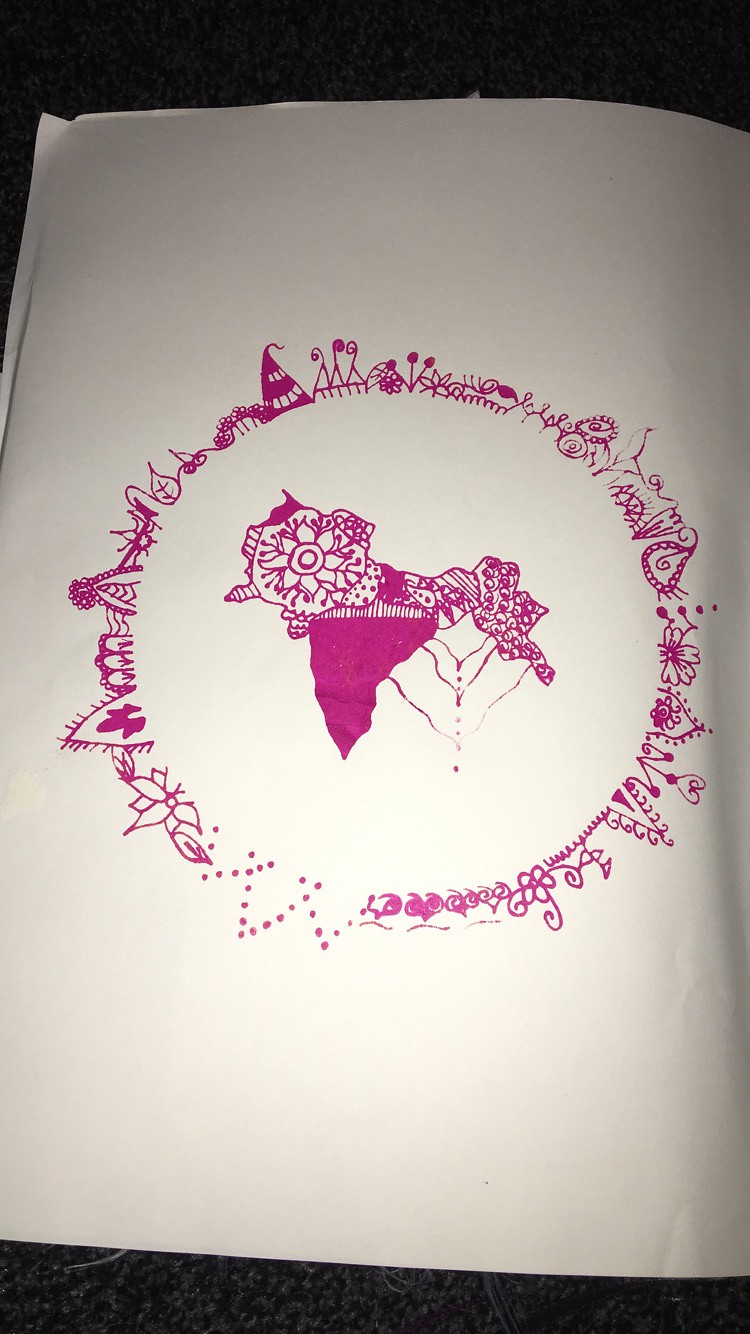This image captures a detailed drawing rendered in pink ink on white sketch paper, positioned on a dark, nearly black tabletop, possibly a countertop. The artwork depicts a central circular figure adorned with a dress, characterized by intricate, swirling patterns. The dress features an outer circular design, embellished with floral motifs and delicate hat-like elements. The overall composition evokes a whimsical, almost fairytale-like scene with fine, swirling lines that resemble grass or vines extending around the central figure. Small portions of the tabletop frame the top and bottom edges of the sketch, providing a contrasting background that highlights the delicate pink drawing.